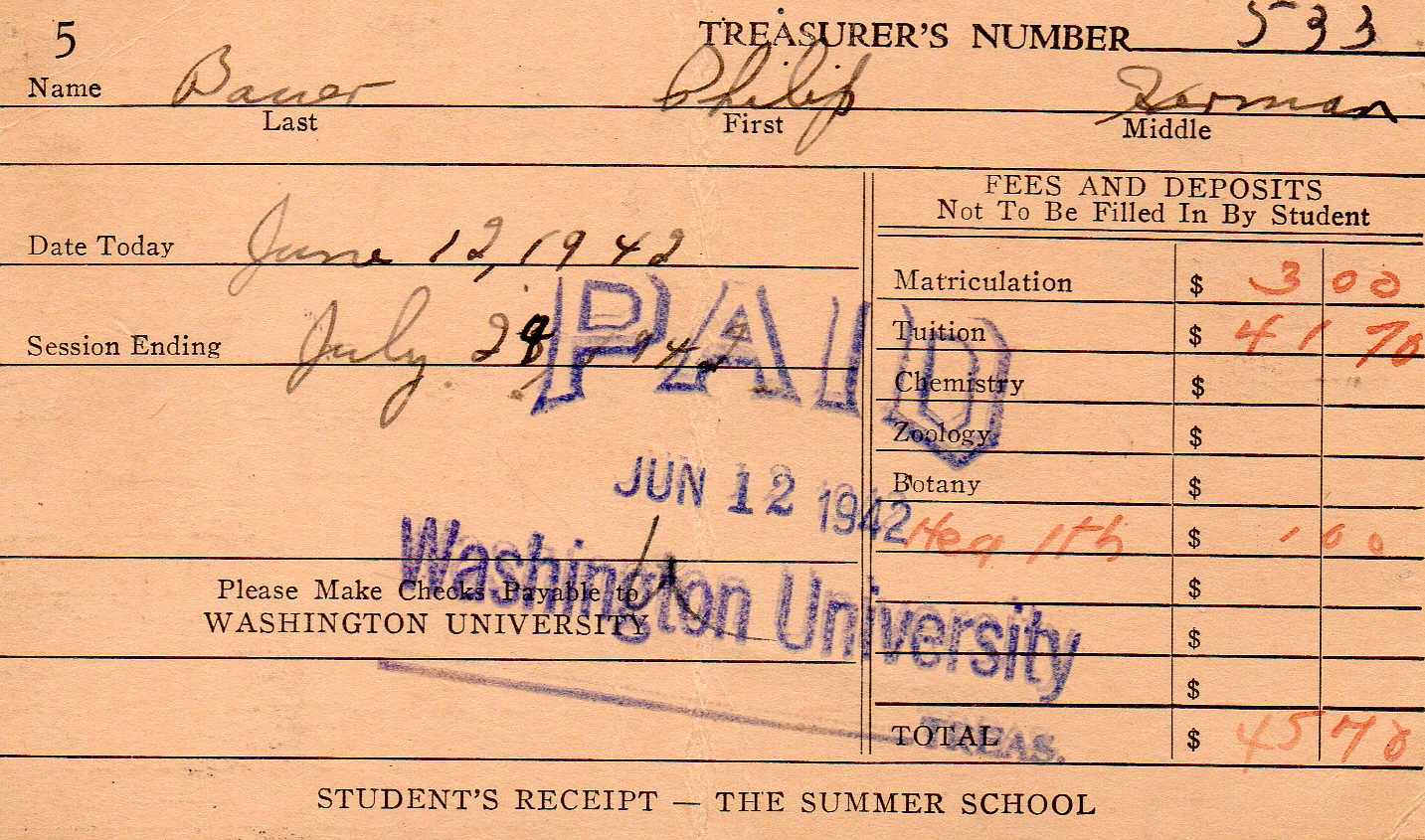This photograph captures an old student's receipt from summer school at Washington University, dated June 12, 1942. The receipt is primarily light pink in color with black font, and includes writing in both light black pen or pencil as well as red pen in some sections. Dominating the top is a blue stamp indicating it was "Paid," dated June 12, 1942. The treasurer's number "533" is noted at the top, and the student's name is written as "Bauer, Philip Herman." The receipt details the date and duration of the session, which ends on July 24, 1942, along with instructions to make checks payable to Washington University. On the right side, it lists various fees and deposits, which are not to be filled in by the student: matriculation fee of $3, tuition fee of $41.70, and a health fee of $1, bringing the total to $45.70. Additionally, subjects like chemistry, zoology, and botany are mentioned. The document appears to be an official invoice or receipt, meticulously filled out and marked paid.